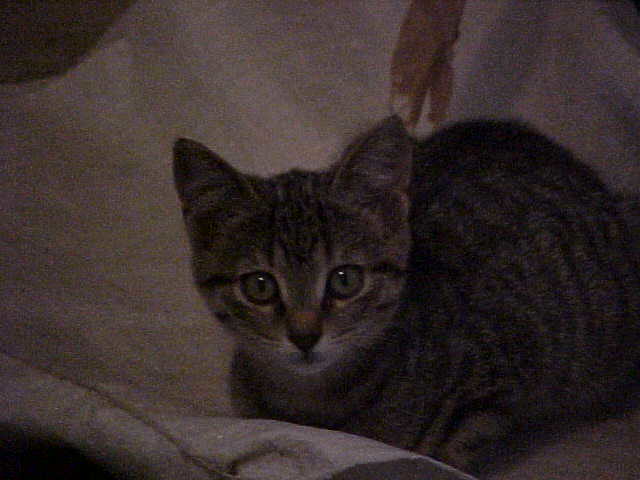This is a vertical rectangular image of a young kitten nestled on a light-colored, possibly white or gray, blanket. The kitten, which has a gray body with black stripes and subtle hints of white, is curiously staring directly at the camera with big, reflective eyes. Its ears are perked up, and it has its legs and paws tucked beneath its body, giving it a crouched appearance as if it is unsure of what might happen next. The background is composed of a gray material that encases the kitten like a soft sackcloth, with the blanket beneath it draped over what appears to be a brown floor or table. There is a noticeable object behind the kitten, though it is unclear whether it's part of the blanket or another indistinguishable item due to the dim lighting of the image. The kitten's whiskers and small facial markings are faintly highlighted, which adds to the charming detail of this dark, shadowy photograph.